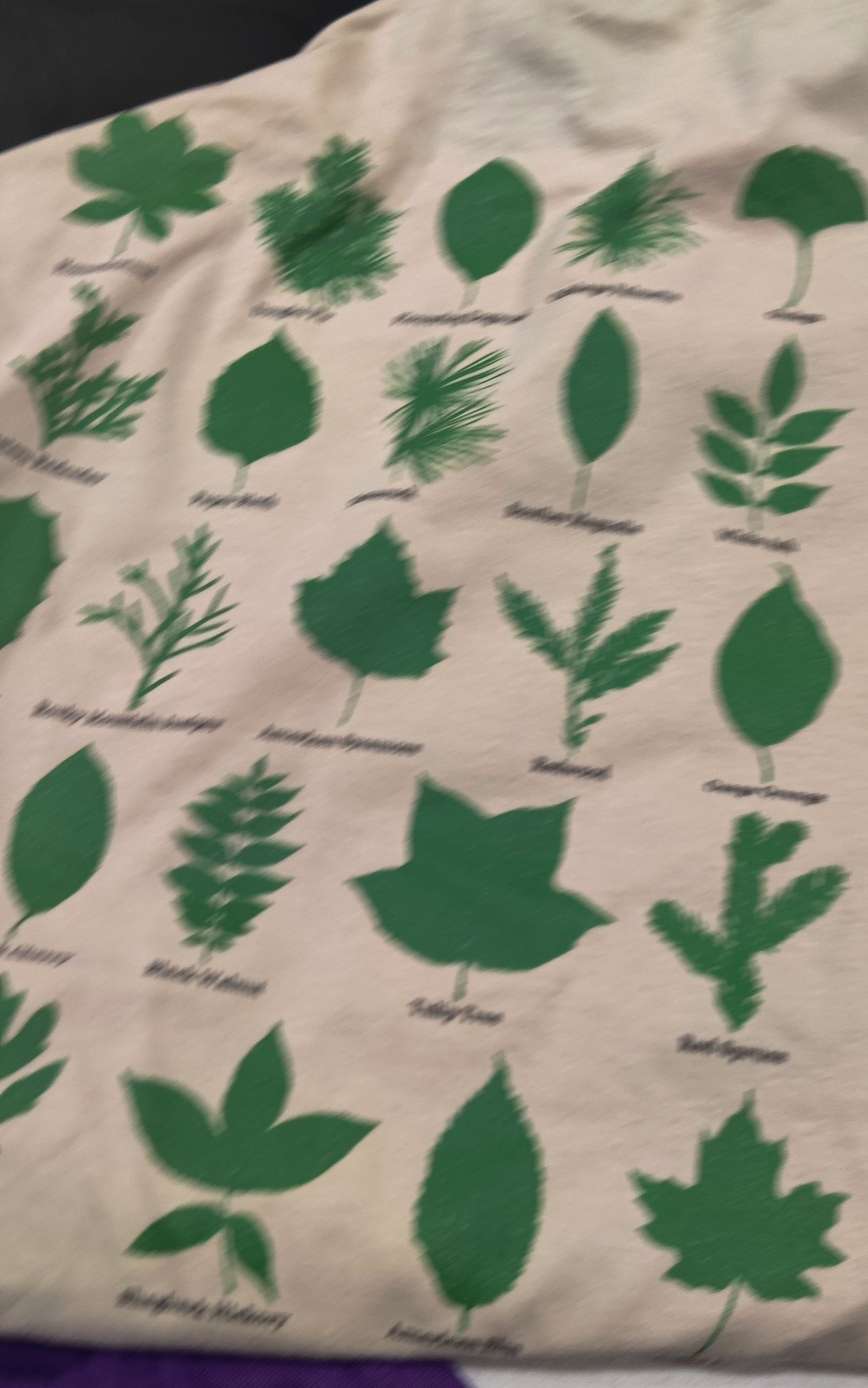This image displays a very blurry photograph of a white cloth or canvas sheet adorned with various green leaves, each accompanied by a black text label underneath. The intense blur makes it challenging to discern the text, leaving the names of the leaves unreadable. The art on the fabric features approximately 20 to 25 different types of leaves, ranging from single leaf structures to those with multiple leaves on a stem. Notably, the leaves are depicted in a dark yet bright green that stands out against the white background. Among the leaves, identifiable types such as pine, maple (located in the bottom right corner), and ash (to the left of the maple) are present. The fabric itself exhibits numerous wrinkles, especially at the top, indicating that it is a soft material. The leaves are arranged in five rows, enhancing the artistic layout on the blurred white cloth.